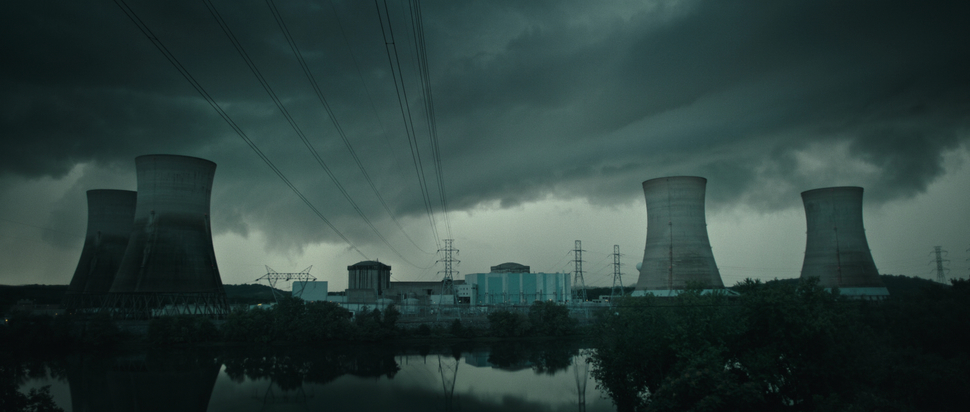The photorealistic image presents a somber and eerie scene featuring an outdoor landscape dominated by a nuclear power plant. Centrally located are four tall, gray cylindrical reactor towers, two positioned on each side of the image. The sky overhead is heavily overcast with dark, menacing clouds that cast a gloomy, gray atmosphere over the entire scene. In the foreground, a large, still body of water mirrors the overcast sky and surrounding low, dark green foliage. Power lines weave from the middle of the image, descending toward the viewer and continuing off the top of the frame. In the distance, a few small gray and blue buildings are visible, adding to the industrial setting. The entire composition, with its heavy clouds and still reflections, amplifies the eerie, near-apocalyptic mood.